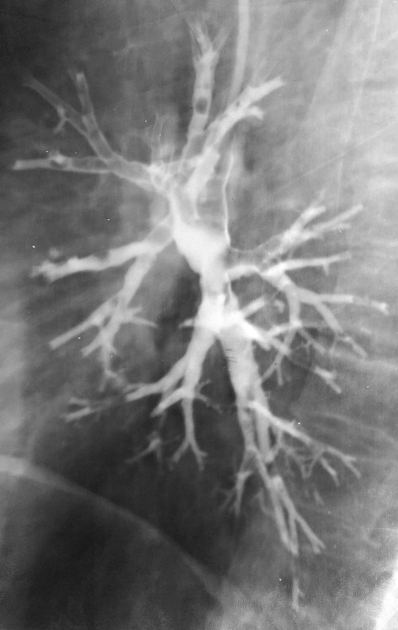This image, rendered in black, white, and shades of gray, appears to be an extreme close-up, almost reminiscent of an x-ray or microscopic view, though its exact nature is unclear. Dominating the scene is a central, ghostly white and gray structure that resembles the form of artery branches or tree roots, characterized by a main stalk in the middle from which numerous branches extend. This structure, which floats unattached against a dark gray background, grows more intricate and thicker towards the top, while tapering and becoming finer towards the bottom. The image is angled so that the top veers towards the top left and the bottom towards the bottom right. Despite a few indistinct details in the background due to the extreme close-up and angle, the primary focus is this intricate, floating, branching form.